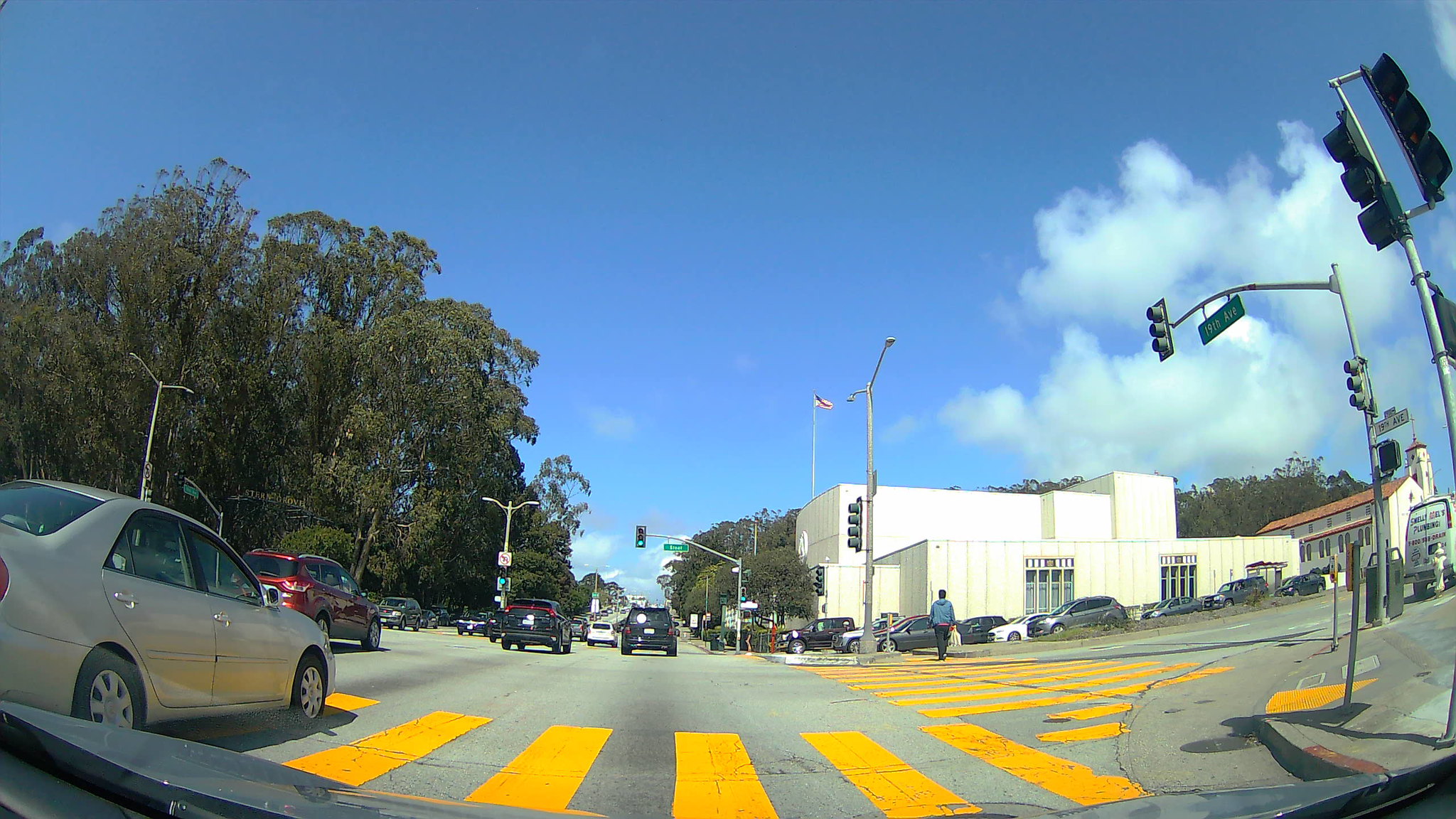This photograph, captured from within a moving car, portrays a vibrant city street scene at a busy crosswalk. The perspective reveals the car's windshield framing the view, with yellow crosswalk lines clearly visible both in front of and to the side of the vehicle. Multiple streetlights dot the background, illuminating the area.

To the right, a prominent white building stands adjacent to a parking lot filled with an assortment of parked cars. On the left side of the image, towering, lush green trees create a canopy over the sidewalk. Only one pedestrian is visible, distinguished by their blue jacket and black pants, walking away from the camera.

In the traffic scene, various vehicles are observed: a tan car to the left, followed by a line of black and white cars. This dynamic snapshot at a streetlight encapsulates the essence of city life, framed by a mix of architecture and nature.